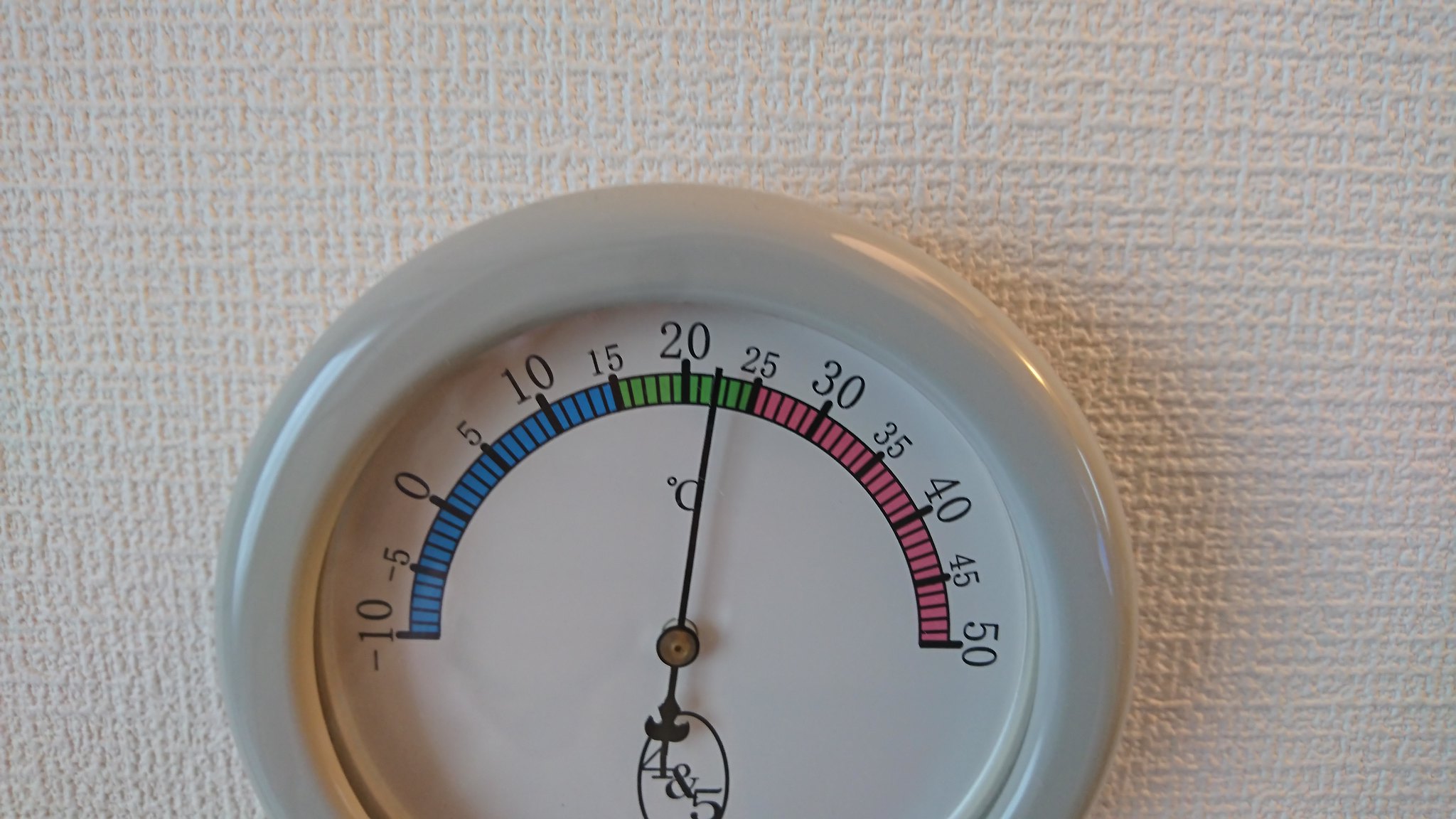This horizontally oriented color photograph features a detailed image of a weight scale, likely a food scale. The scale is crafted with a circular face encased in light gray plastic or ceramic material. The exterior ring evokes the design of a speedometer. Placed on a cross-textured surface resembling thick watercolor paper, the dial's interior is predominantly white with a circular scale around its edge. The scale is marked with numerical increments including -5, 0, 5, 10, 15, 20, and up to 50. Segments of the dial are colored in blue, green, and pink. In the center, a pointer with a delicate leaf design on one end and a straight tip on the other, is anchored by a bronze screw. Below the leaf design, within an oval, the numbers "4 5" are printed in black text.